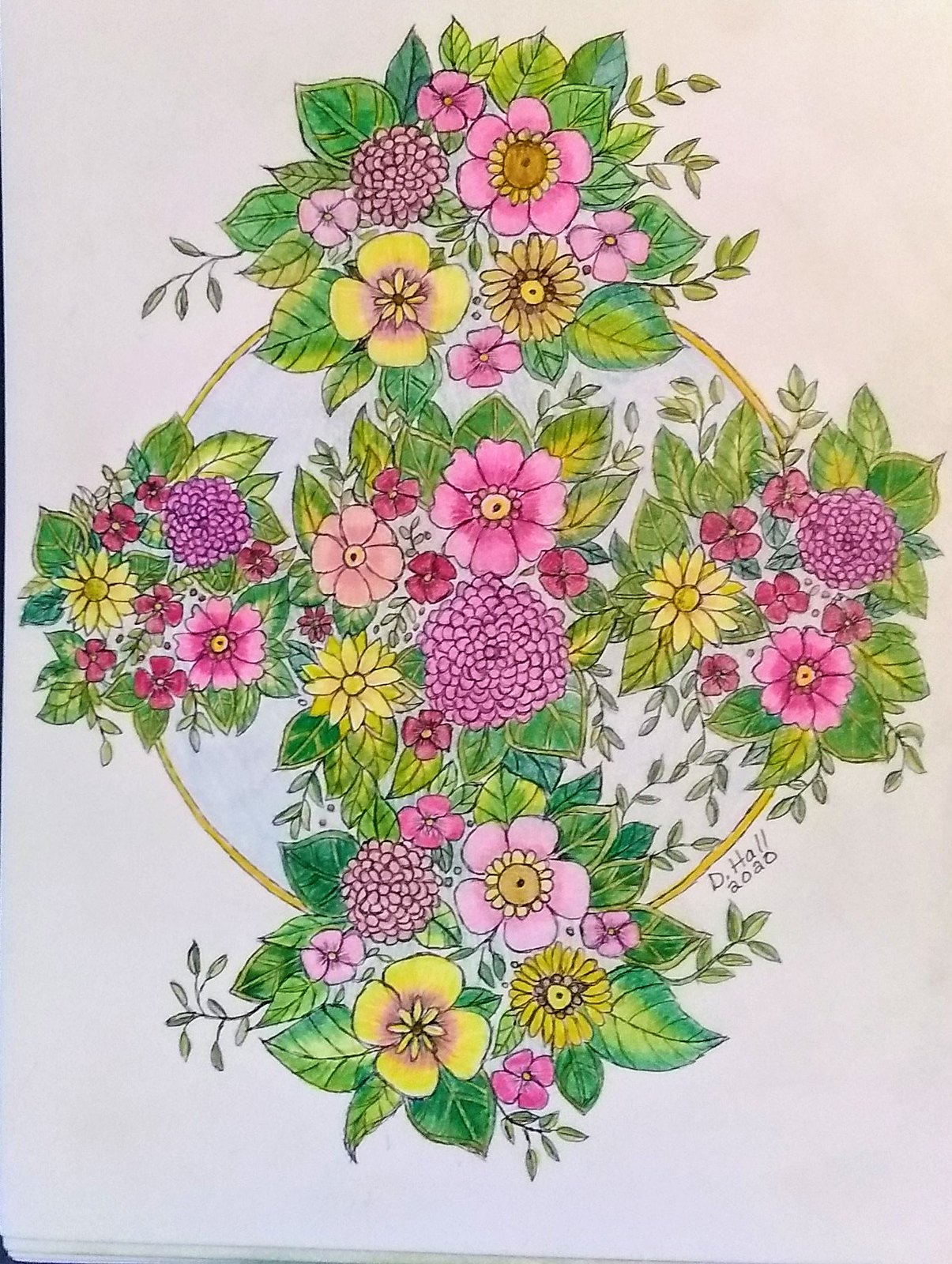This intricate drawing, completed in 2020 by D. Hall, features a vibrant floral theme, meticulously arranged around a central gold circle. Encircling the golden centerpiece are elaborate flower motifs positioned at the top, bottom, left, and right. The composition showcases predominantly bold pink petals with yellow centers, interlaced with alternating yellow petals with pink centers, creating a harmonious color scheme throughout the piece. Behind the flowers, lush green leaves add depth and contrast. At the bottom of the artwork, numerous small circles outlined in black and filled with pink form a cluster, resembling a gathering of delicate blooms. The artist's signature, "D. Hall 2020," is subtly placed on the right side, underscoring the creator's identity.